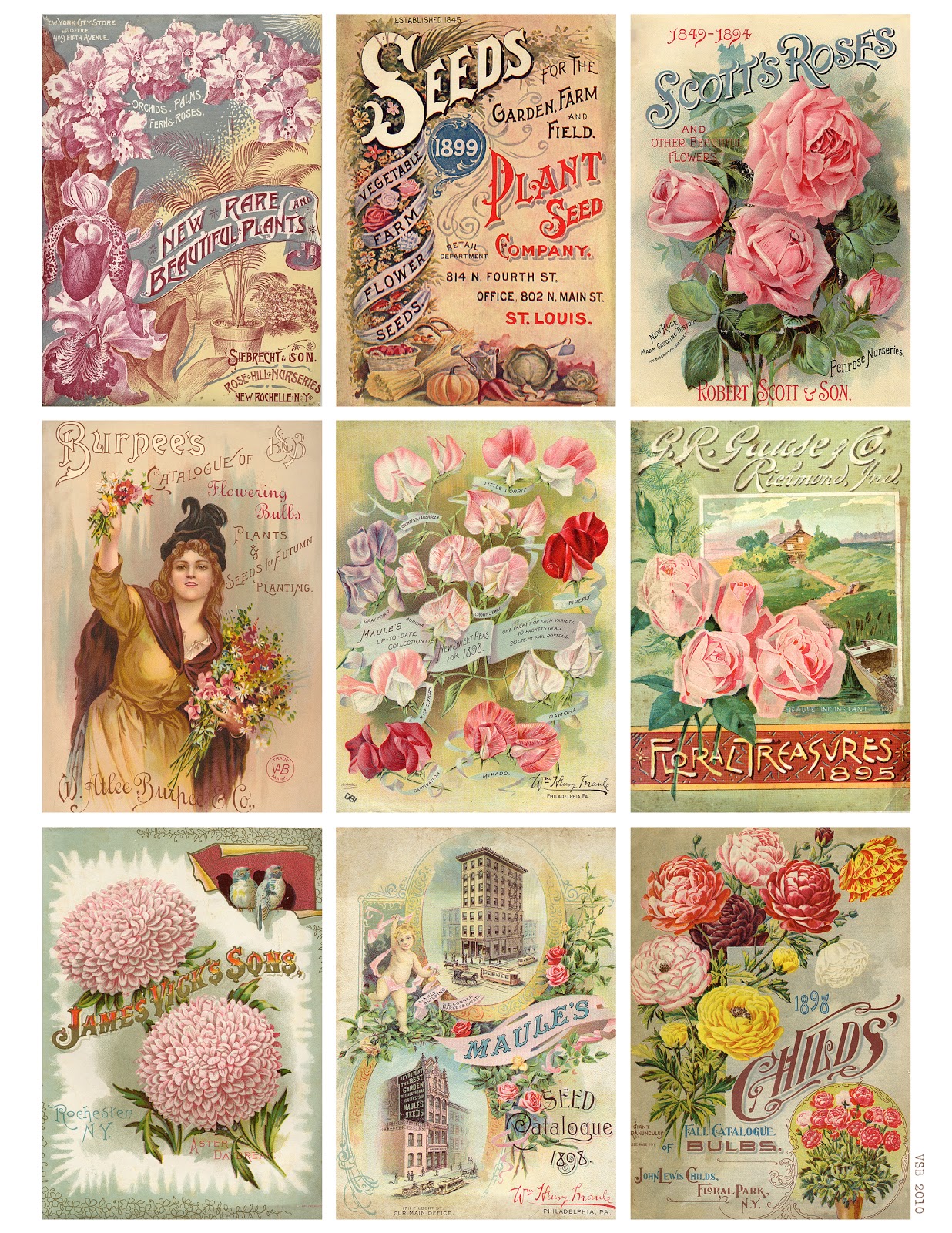The image showcases a vintage-inspired poster featuring nine individually styled seed packets arranged in three rows of three. Each packet prominently displays various flowers, with a consistent emphasis on pink blossoms. Among the assortment of flowers depicted, other hues like red, yellow, and purple make an appearance, yet the pervasive theme remains pink flora. The packets exhibit an old-style Americana or Victorian aesthetic, suggesting an era around the late 19th to early 20th century, some marked with dates like 1849 to 1899.

The top left packet announces "New Rare Beautiful Plants" adorned with a variety of pink flowers. Adjacent to it, another packet with a cream background lists "Seeds for the Garden Farm Enfield Plant Seed Company," hailing from St. Louis, stamped with the year 1899. The top right packet foregrounds vibrant pink roses under the heading "Scott's Roses, 1849 to 1894," attributed to Robert Scott and Son.

In the middle row, the leftmost packet features a light-skinned Victorian lady in a gold dress and black hat, holding large bouquets of flowers in both hands. The intricate designs of these packets reflect the classic, muted color palette typical of the era's printing.

Overall, every packet on this poster emanates an antiquated charm, celebrating the timeless beauty of flowers like roses and wildflowers, with nostalgic imprints such as "Burpee Seeds" and "Child Seeds" adding to the historical allure. The detailed depictions and faded coloring combine to create a cohesive, visually pleasing homage to a bygone botanical advertising era.